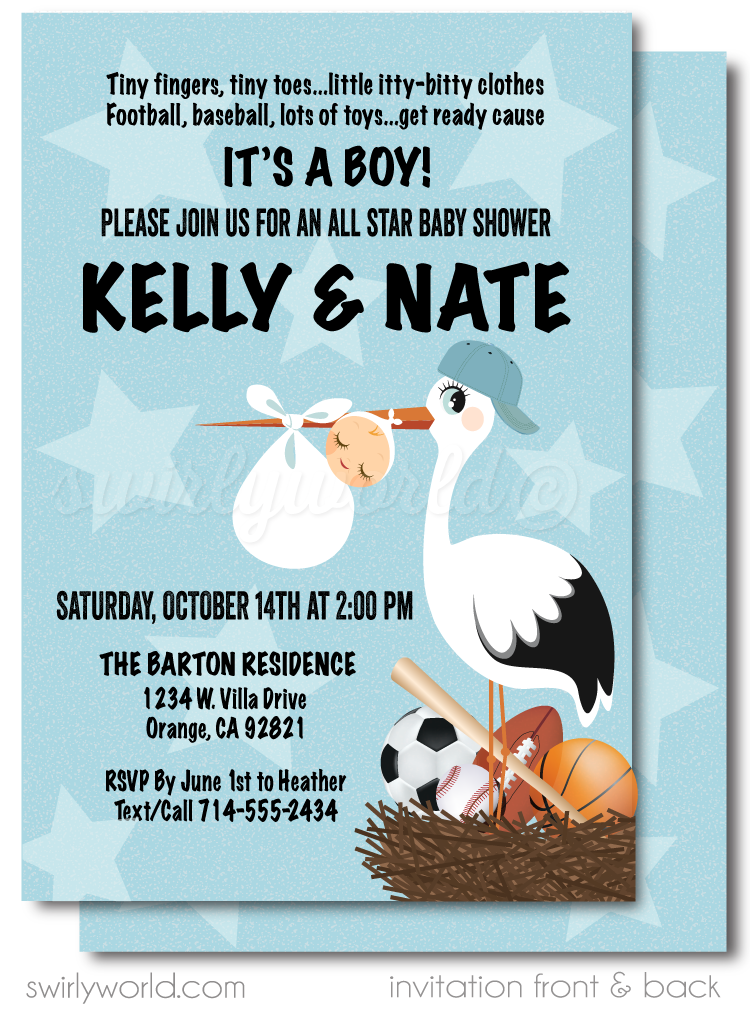The image depicts a computer-generated blue invitation card adorned with light blue stars around the border. At the top in black letters, it reads, "Tiny fingers, tiny toes, little itty-bitty clothes, football, baseball, lots of toys, get ready 'cause it's a boy. Please join us for an all-star baby shower for Kelly and Nate." Below this cheerful announcement, a stork wearing a blue backwards cap is illustrated, carrying a bundled baby at its beak. Adjacent to the stork, a small basket brimming with various sports equipment—soccer ball, baseball, football, and basketball—adds a playful touch. The event details are clearly listed on the bottom left, "Saturday, October 14th at 2 p.m. The Barton Residence, 1234 West Villa Drive, Orange, California, 92821." Further instructions to RSVP by June 1st to Heather via text or call, with the phone number 714-555-2434, are also provided. The entire invitation is credited at the bottom to “swirlyworld.com,” indicating it showcases both the front and back design of the card.